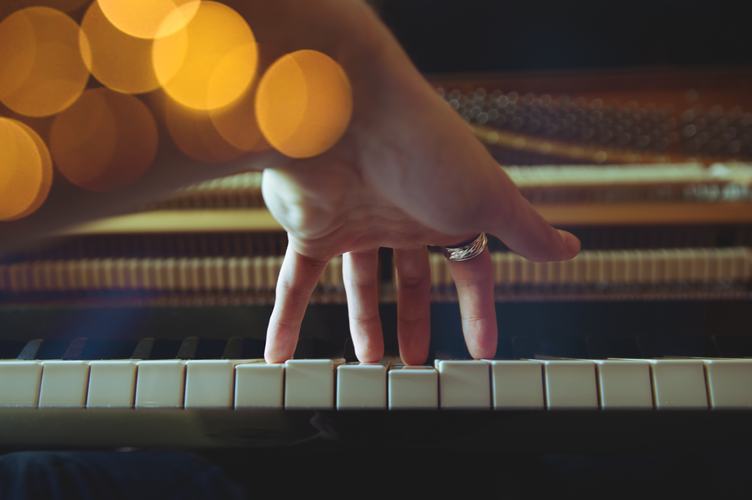The photorealistic image captures a close-up view of a Caucasian hand pressing down on piano keys with four fingers, all except the thumb. The hand, adorned with a silver ring on the pointer finger, extends from the top left corner of the frame. The piano stretches horizontally across the image from right to left. The camera angle focuses on the sides of the keys, displaying approximately two octaves’ worth of white keys while black keys are visible in the background. The backdrop of the image is slightly out of focus, featuring a mix of indistinct brown, tan, and beige lines that could be part of the piano or something further away. There are also gold-colored lens flares or photographic effects, resembling small sunspots or moons, particularly prominent in the top left corner and overlapping with the hand. The piano's surface appears to have a fabric covering, and beyond the keys, the background fades into darkness.